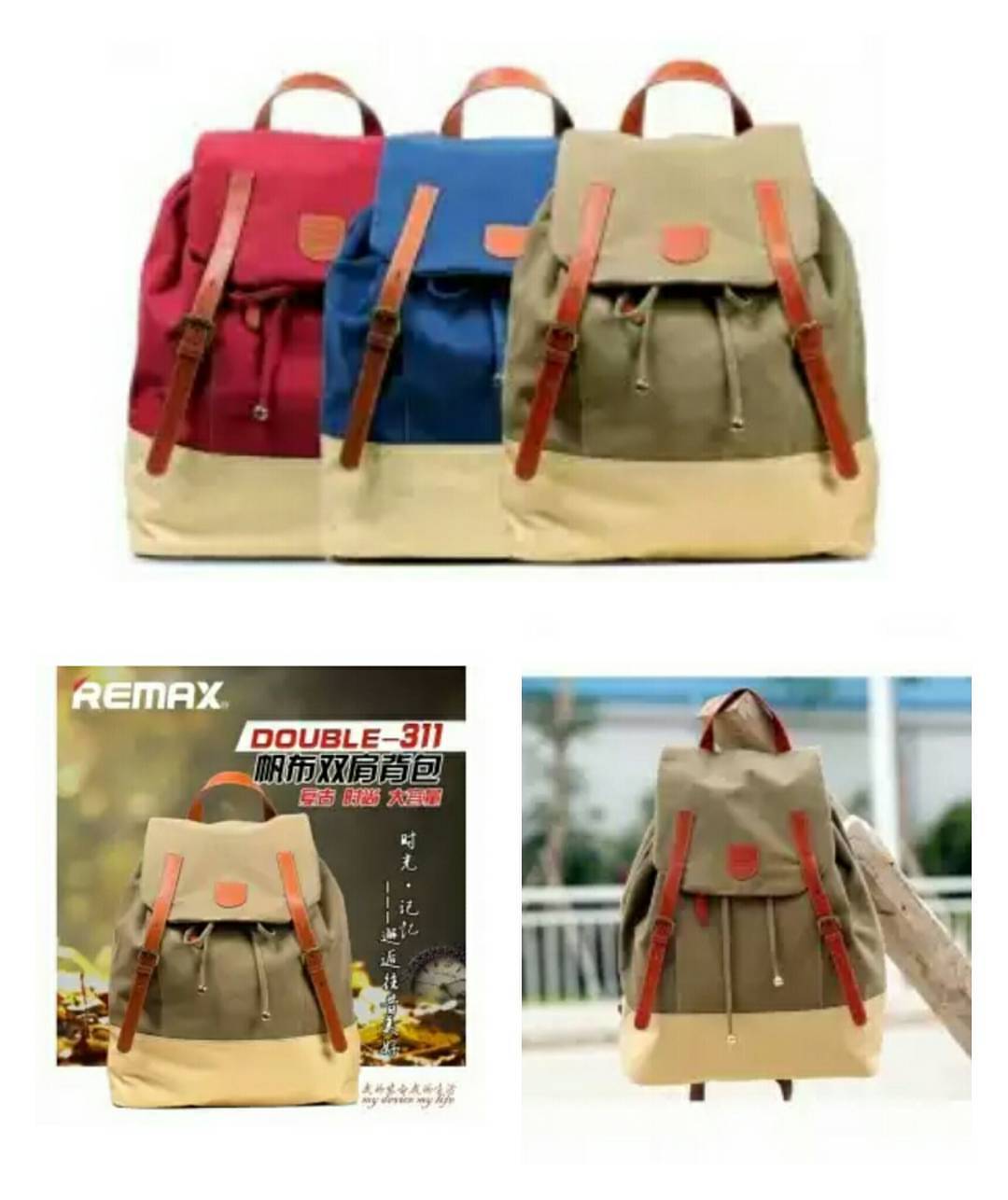This advertisement image features a stylish collection of backpacks arranged in three distinct sections. At the top, three backpacks of identical design but different colors - red, royal blue, and olive green - are showcased. Each bag boasts a beige base, tan drawstrings, and a distinctive flap with brown leather straps and metal buckles for secure fastening. At the very top, the brand name "REMAX" is prominently displayed, along with its logo.

The bottom section is divided into two parts, separated by a small gap. On the left, an image highlights the olive green backpack with corresponding Chinese text, and the English phrase "double dash three one one." The REMAX logo appears in white. On the right, the same olive green backpack is elegantly hung against a wooden panel, emphasizing its practical and trendy design. This comprehensive layout effectively emphasizes the variety in color options while maintaining a consistent, detailed design for potential buyers.